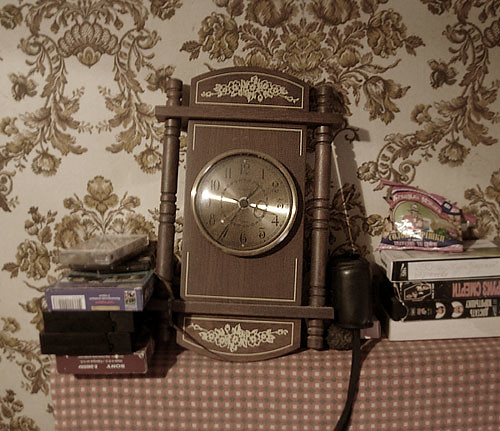The image showcases a photograph of an antique-looking wooden clock, prominently displayed as the main subject. The clock features two intricately designed wooden spindles running along its top and left side, with horizontal wooden panels at the top and bottom, and an additional wooden plank in the middle. The clock's face, in the center, is a golden yellow color with a metallic sheen, displaying the numbers 1 through 12, and is adorned with ornate gold floral patterns at both the top and bottom of the dial. The time displayed on the clock is 1:35.

The clock is positioned on a table draped with a brown and tan checkered tablecloth. Surrounding the clock are various items, including VHS tapes, cassette tapes, a camera, and a bag that appears to contain candy, contributing to a sense of miscellaneous clutter. The backdrop features wallpaper with a cream-colored base and a tan floral design, evoking a vintage aesthetic from the 1970s.